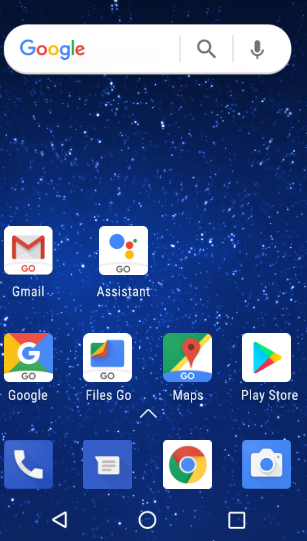This is a screenshot of a mobile browser interface with a Google-themed background. At the very top, there is a Google search bar prominently displayed against a backdrop of a starry night sky. To the right of the search bar, there is a vocal search icon depicted as a microphone and a visual search icon illustrated as a microscope.

Below the search bar, there are ten apps arranged in three rows. The top row features two applications: Gmail on the left and Google Assistant on the right. The second row displays four apps: Google Go, Files by Google, Google Maps, and the Google Play Store, listed sequentially from left to right. The bottom row also contains four apps: a telephone icon for making calls, a note icon representing a note-taking application, the Google Chrome browser icon, and a camera icon on the far right for taking pictures.